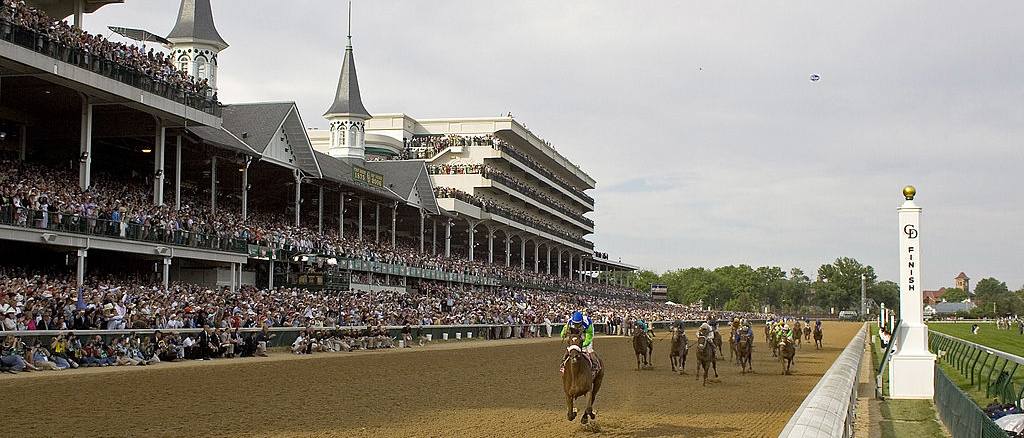The image is a detailed portrayal of the Kentucky Derby at Clover Downs on an overcast day, capturing the excitement as the horses come across the finish line. The focus is on a brown lead horse, ridden by a jockey in a neon orange attire paired with a blue helmet, significantly ahead by several horse lengths of the trailing pack. The stands are completely full with spectators in their Derby Day wear, with additional viewers observed on the green field and even on the roof, all absorbed in the race. Professional photographers are strategically seated alongside the track, ensuring an unobstructed view for the audience. The grandstand structure is extensive, featuring multiple tiers — two main rows and an attic row on one side, with three additional ascending sections at the far end, all packed with eager fans. The image beautifully captures the essence and vibrant atmosphere of this prestigious event.